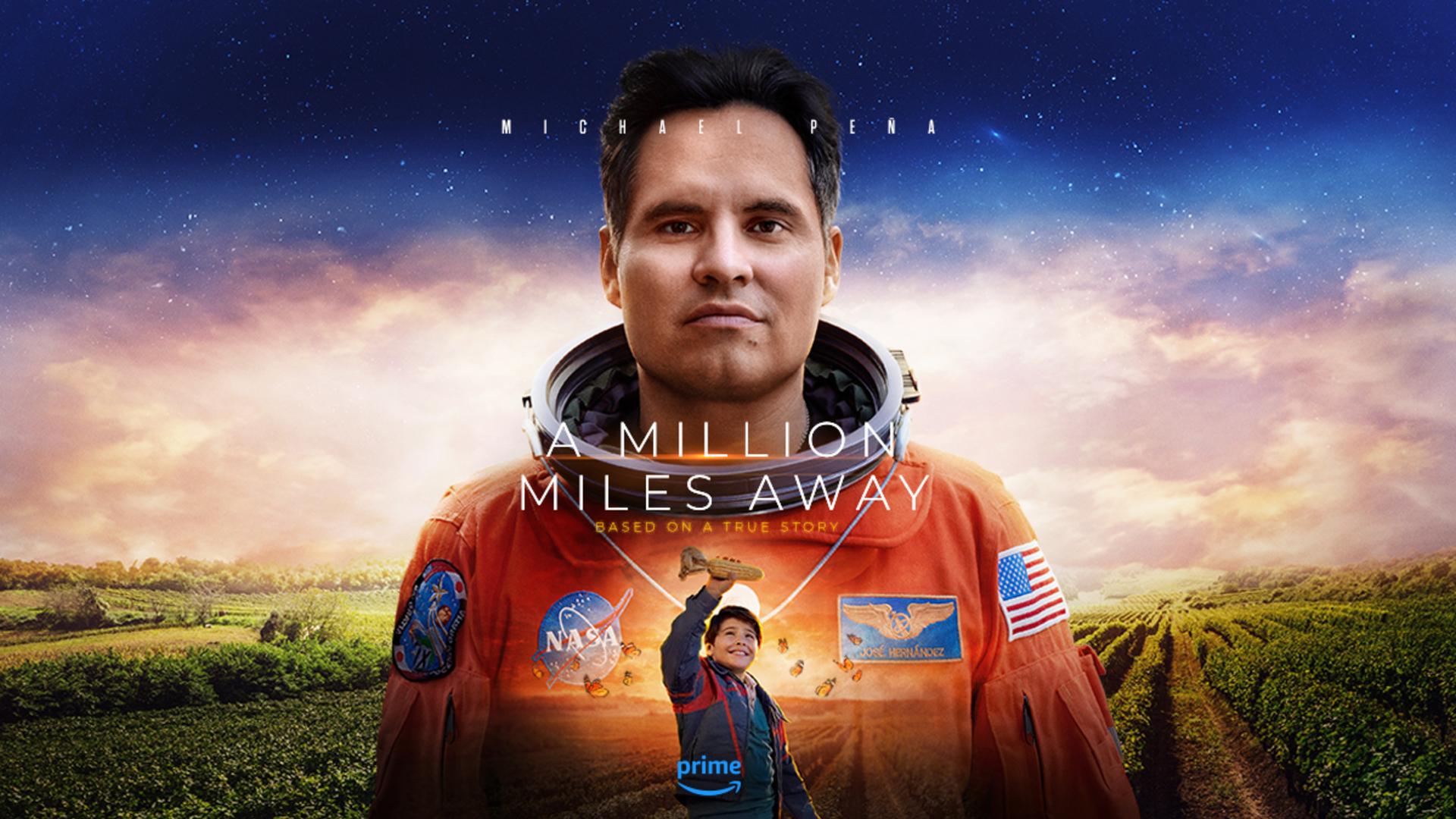This vibrant movie poster, set in a horizontal rectangle, features prominent actor Michael Peña at its focal point. His name, "Michael Peña," is emblazoned in white uppercase letters across the top of the image. Peña, depicted in a detailed NASA spacesuit, stands with a stern expression. His dark, short hair and brown eyes contrast with the spacesuit's bright orange color. The suit features several notable patches: a blue patch with a bird on his right chest, the NASA logo on his left chest, an American flag on his right shoulder, and an indeterminate blue patch on his left shoulder. The most striking part of his suit is the large brown collar intended for a helmet attachment.

Centrally displayed in white text across his chest is the phrase "A Million Miles Away," with some smaller, unreadable text beneath it. Superimposed over Peña's image is a smaller figure of a boy in a blue jacket with red stripes, joyfully holding up a wooden airplane above his head, gazing at it with a smile. This boy's depiction includes the word "Prime" in blue letters with a circular arrow beneath it across his midsection.

The background showcases lush, green farmland with orderly rows of crops that gradually transition into a dramatic sky. The upper part of the sky is a deep blue speckled with white stars, while lower down, it turns into a blend of clouds illuminated by purple and pink sunlight. This rich and colorful backdrop reinforces the grounded yet aspirational theme of the movie advertised in this compelling poster.